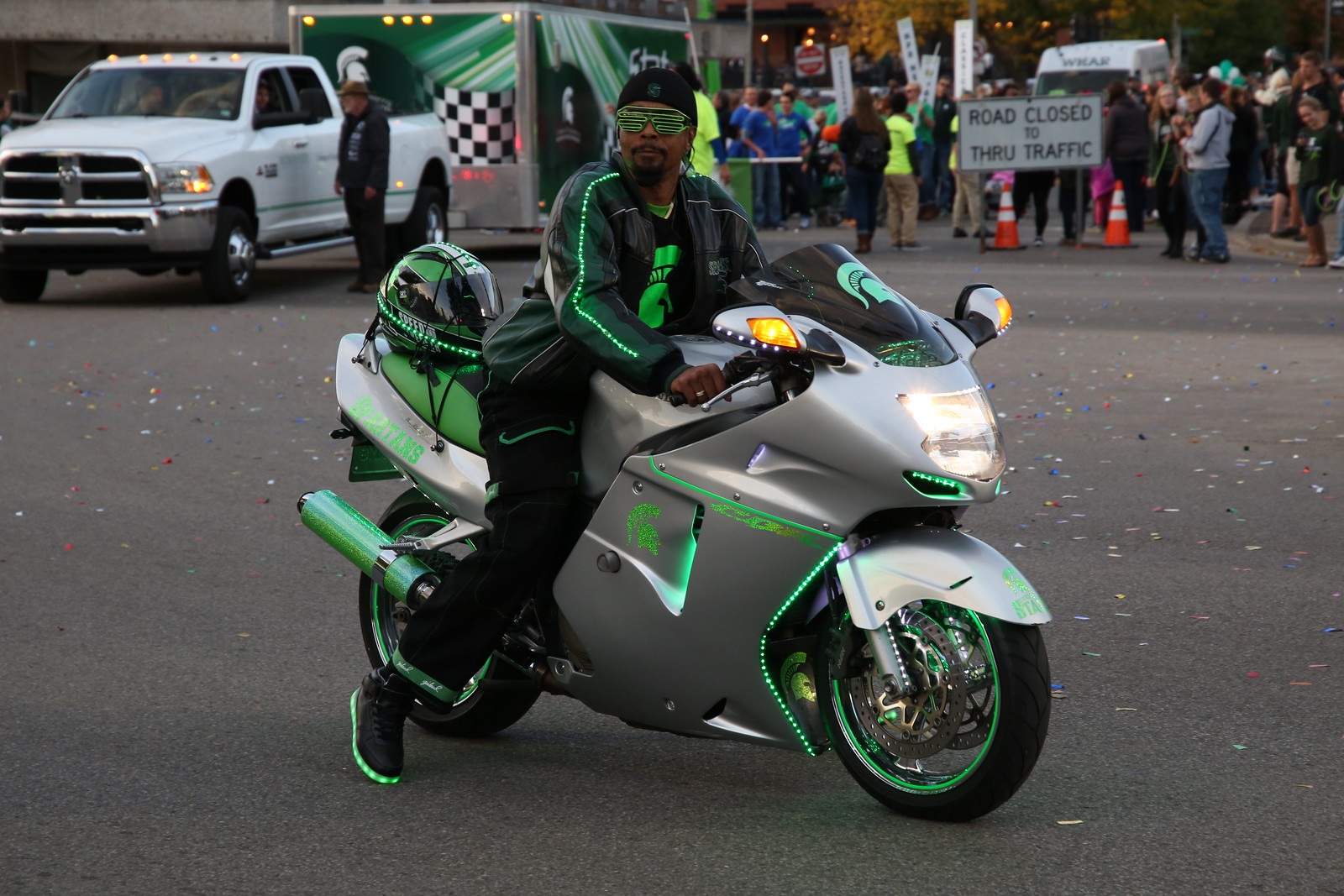In this detailed outdoor scene set during the middle of the day, a striking photograph captures a man of African descent positioned directly in the center, sitting on a futuristic-looking silver motorcycle accented with green neon lights. He is dressed entirely in black with coordinated green elements, such as a black leather jacket with green pinstriping and illuminated features, black pants with green cuffs, and black shoes with green soles. Sporting green sunglasses and a black cap turned backward, he has a mustache and a chin beard, and an additional black t-shirt adorned with a bright green logo is visible beneath his open jacket.

The motorcycle, detailed with green neon lights on the rims, highlights, and tailpipe, shines under the daylight. The leather seat is also characterized by its neon green hue, emphasizing the bike's modern aesthetic. The motorcycle's headlights are turned on, revealing graffiti-like confetti scattered on the gray asphalt road beneath.

In the upper part of the image, a bustling crowd is contained by orange traffic cones and a "Road Closed to Through Traffic" sign. A white Ram pickup truck towing a large, enclosed green and silver motorcycle trailer with a checkered flag design is visible beyond the man. The truck is engaged in conversation with individuals at a checkpoint. This suggests an event ambiance, possibly a parade or public gathering, held on the closed-off street, with various colors such as gray, black, green, silver, orange, yellow, blue, and white subtly enriching the scene.